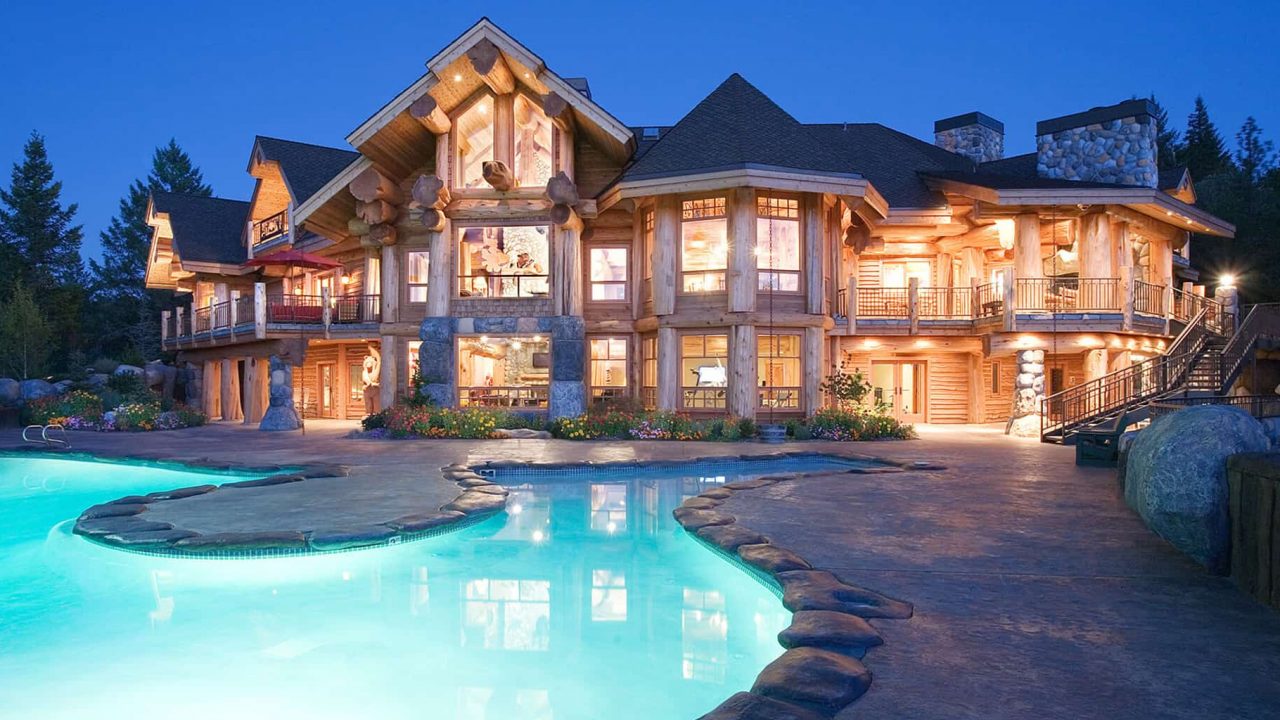The photograph captures a grandiose log cabin mansion, evoking a sense of luxury and tranquility. Dominated by large exposed beams and two prominent stone chimneys, the mansion stands majestically against an evening sky that transitions into deep indigo blue. The home is brilliantly illuminated from within, casting a warm golden glow that highlights its intricate architectural details, including a pointed, column-like section with a sharply sloped roof.

Spanning three stories in the center with two-story wings on either side, the mansion features expansive balconies running the length of the upper floors, offering a panoramic view of its surroundings. The reflection of the illuminated house shimmers in the adjacent swimming pool, which curves in a U-shape and features an island and decorative rocks around its edge. The pool, glowing a mesmerizing teal, extends from the right side of the photograph towards the viewer, bordered by stone tiles.

The surrounding area is lush with trees that frame the mansion and enhance its secluded ambiance. The patio area leads seamlessly into the pool, inviting relaxation and outdoor enjoyment. This breathtaking scene is a harmonious blend of natural beauty and architectural splendor, making the mansion appear as a luxurious retreat nestled in a picturesque setting.